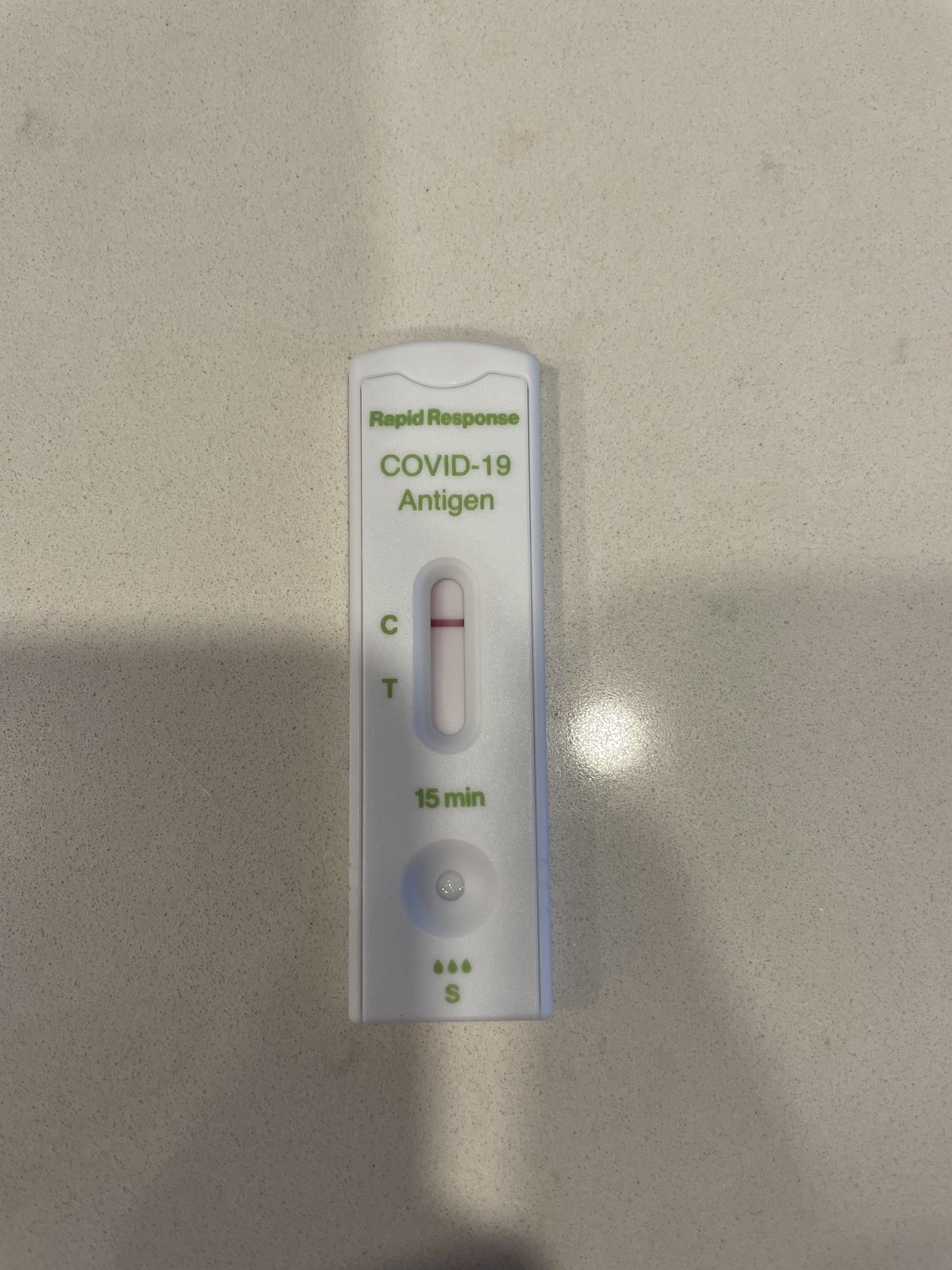An out-of-focus photograph captures a COVID-19 rapid response test device positioned on a white surface. Dominating the center of the image is a bright reflection, likely from a flash or overhead light, possibly originating from an iPhone used to take the picture. The photograph features two prominent shadows from the iPhone, one on the right and one on the left, extending across the bottom half of the frame.

The test device, centrally located, prominently displays the text "Rapid Response COVID-19 Antigen" in green. Adjacent to an oval-shaped window on the device are the letters "C" and "T," with a red line visible next to the "C." Below this window, the text "15 min" is indicated. Near the bottom of the test device, there is a designated area marked with an "S," accompanied by three drop icons, suggesting where to deposit the sample drops.